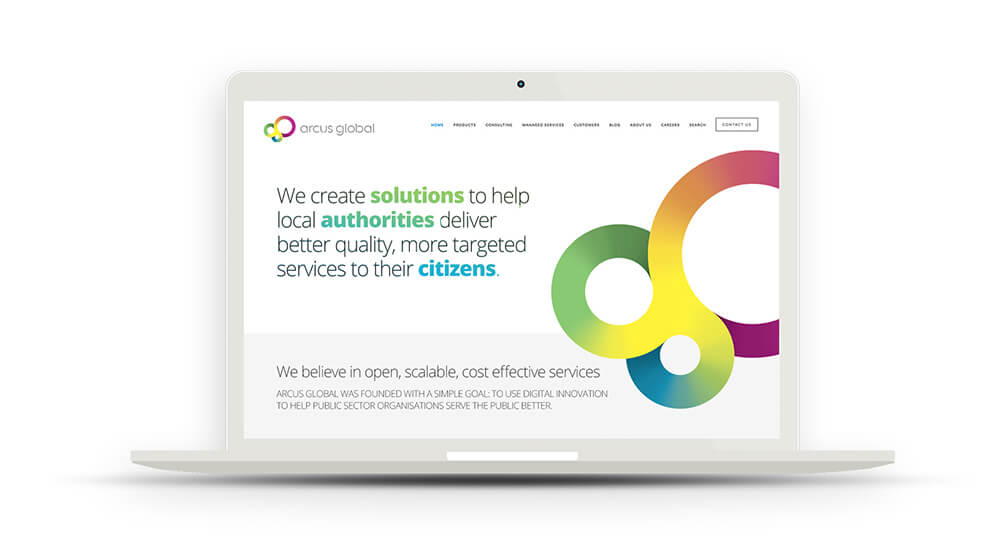This is a highly detailed mock-up image of a website displayed on a minimalist, futuristic-looking laptop. The laptop, appearing almost artificial in its immaculate cleanliness, is completely white, and strikingly devoid of any physical keyboard. The only visible features are the bottom edge and top bezel framing the screen, alongside a single front-facing camera. The laptop itself is beige, contributing to its understated, almost sterile aesthetic.

The website on display occupies the entirety of the screen, without any accompanying taskbar or navigation bar, suggesting the image might be purely a graphical representation rather than a functional interface. The website belongs to "Arcus Global," a company dedicated to creating innovative solutions to enhance the quality and specificity of services provided by local authorities to their citizens. The company's philosophy centers around open, scalable, and cost-effective services.

An abstract, emblematic icon representing Arcus Global is prominently placed, consisting of three interlocking circles that converge in the middle. Each circle has a gradient that merges into a central yellow core. The largest circle transitions from red to yellow, the medium circle from dark green to yellow, and the smallest circle from blue to yellow, creating a visually captivating and complex logo.

At the top of this mock-up webpage, there are nine tiny menu icons, so diminutive that their labels are illegible, suggesting they could be placeholders or simply decorative elements. Despite their insignificance in size, their presence adds a layer of realism to the mock-up, hinting at the comprehensive nature of the website's intended design.